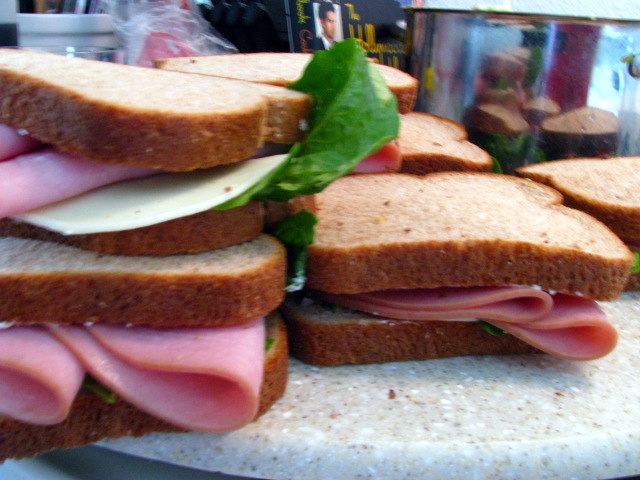The image depicts a horizontal arrangement of sandwiches on a circular, granite-like countertop with an off-white coloration and tiny beige dots, possibly resembling ceramic. The sandwiches are mostly composed of whole wheat or whole grain bread with brown crusts, filled predominantly with folded slices of pink ham. Among them, the sandwich in the foreground shows wheat bread, several slices of ham, a spread of mayonnaise, and possibly some lettuce peeking beneath the meat. Another prominent sandwich to the left includes white cheese, likely Swiss or American, a green leaf of lettuce, and the same type of ham, all between two slices of bread with brown crusts. Additionally, several sandwiches are stacked toward the back, partially obscured but indicated by their visible crusts. In the background, there’s a white ceramic cup holding items that seem to be pens, a clear cup, a black picture frame or brochure with a man's photo, and a clear case containing undetermined objects. The overall scene suggests a kitchen setting, and the reflective metallic surface behind the sandwiches adds depth to the composition.